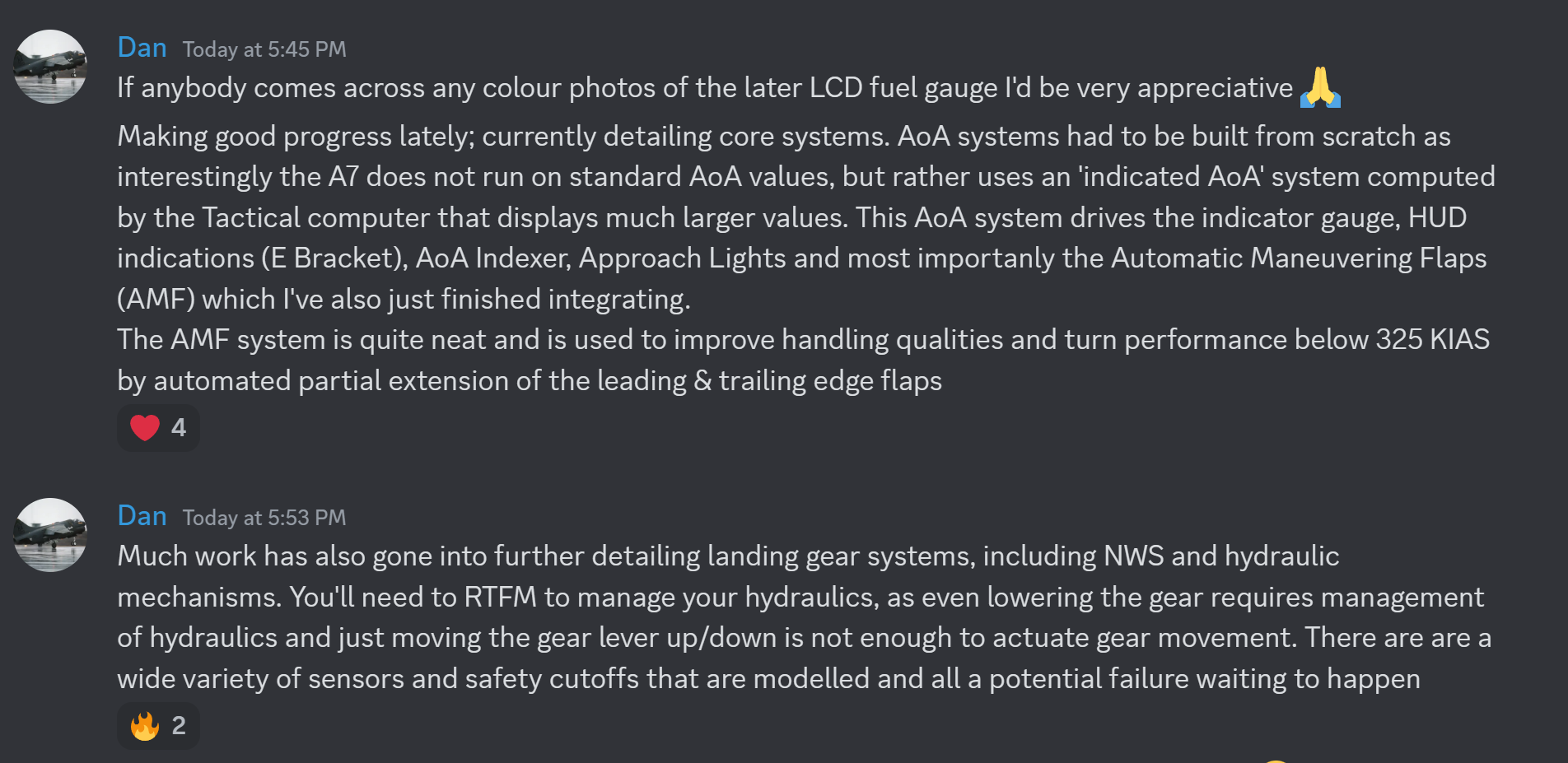**Post by Dan, Today at 5:45 PM:** 

*Detailed Update on A7 Systems with Image Request*

I am making good progress lately with core systems, and I am currently focusing on detailing. The AOA (Angle of Attack) systems had to be entirely rebuilt from scratch. Interestingly, the A7 does not operate on standard AOA values but uses an indicated AOA system computed by a technical computer, which displays significantly larger values. This AOA system controls an array of indicators and systems, including the indicator gauge, HUD indicators, E-bracket, AOA indicator, approach lights, and, most importantly, the automatic maneuvering flaps (AMF). 

I have also finished integrating the AMF system, which is designed to improve handling and turn performance below 325 knots indicated airspeed (IAS) by partially extending the leading and trailing edge flaps automatically.

Additionally, much work has been put into further detailing the landing gear systems, including nosewheel steering (NWS) and hydraulic mechanisms. Managing hydraulics is crucial, as even lowering the landing gear requires careful management. Simply moving the gear lever up or down is insufficient to actuate gear movement. There are various sensors and safety cutoffs modeled, each a potential failure waiting to happen.

**Likes**: 4 ❤️

**Request**: If anyone comes across any color photos of the later LCD fuel gauge, I would be very appreciative. 🙏

[Blue background indicating this is a visually formatted post]